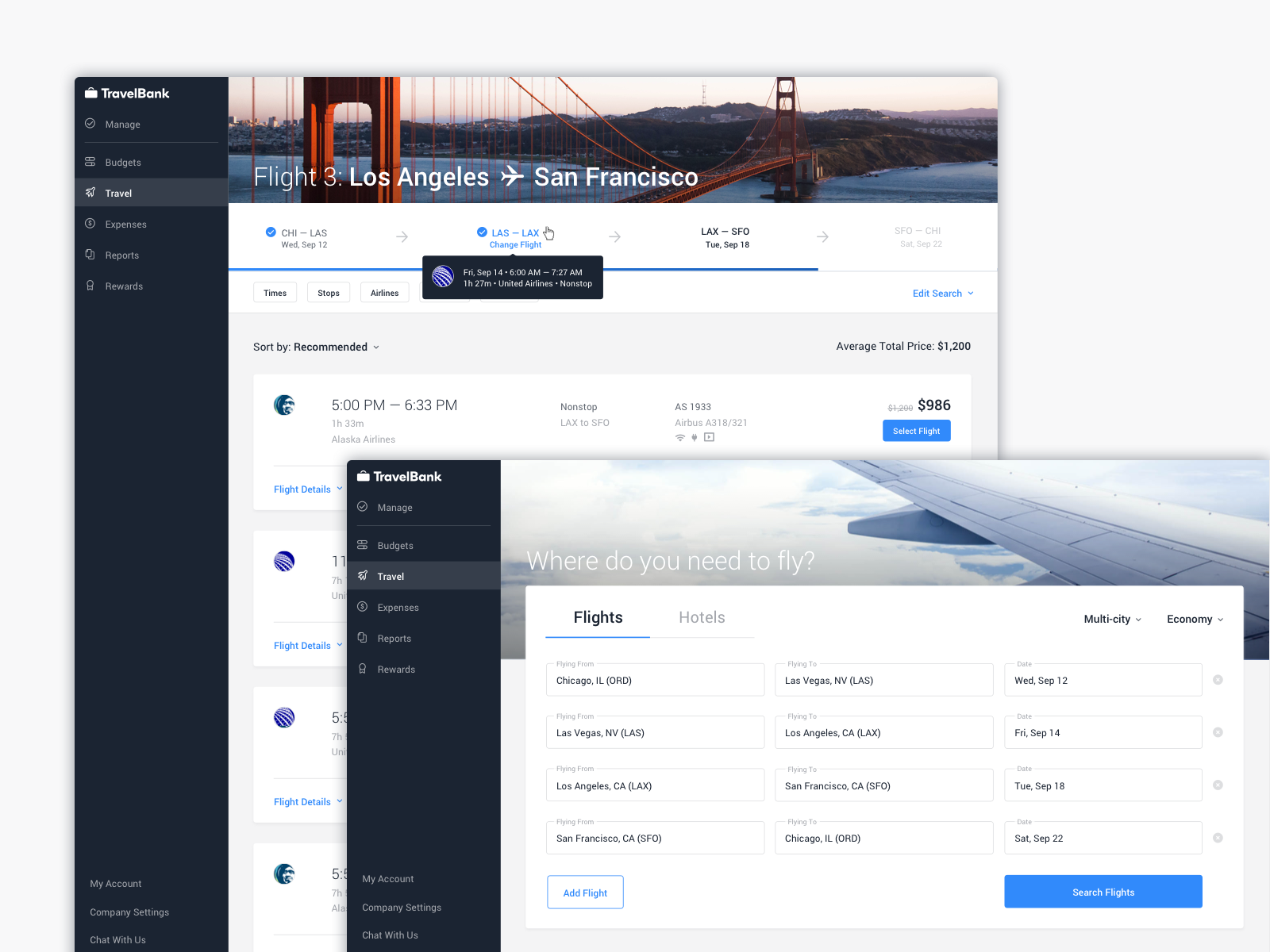**Detailed Caption:**

This image is a screenshot of a multi-flights booking application displaying two separate windows. 

In the first window, there are two distinct panels. The left panel is narrow and features "Travel Book" at the top, followed by a list of options starting with "Manage Travel," though the remaining items are too small to discern. The right panel prominently displays a header image of the iconic Golden Gate Bridge in San Francisco. Below this image, the title reads "Flight 3: Los Angeles to San Francisco," indicating that the page shows the itinerary details for flights from Los Angeles to San Francisco on a specific date. The first flight option is listed as departing between 5:00 PM and 6:33 PM, starting at a price of $986.

In the second window, also from the Travel Bank website, the overall browser design is consistent with the first window. The title asks, "Where do you need to fly?" In the middle of this window, there's a chart featuring options for both flights and hotels. Additionally, there is a prominently placed drop-down menu with options for "Multi-City" and "Economy." This window lists approximately five or six selectable options.

Overall, the screenshot provides a comprehensive view of flight options and details for users planning trips, emphasizing both single-route and multi-city travel accommodations.